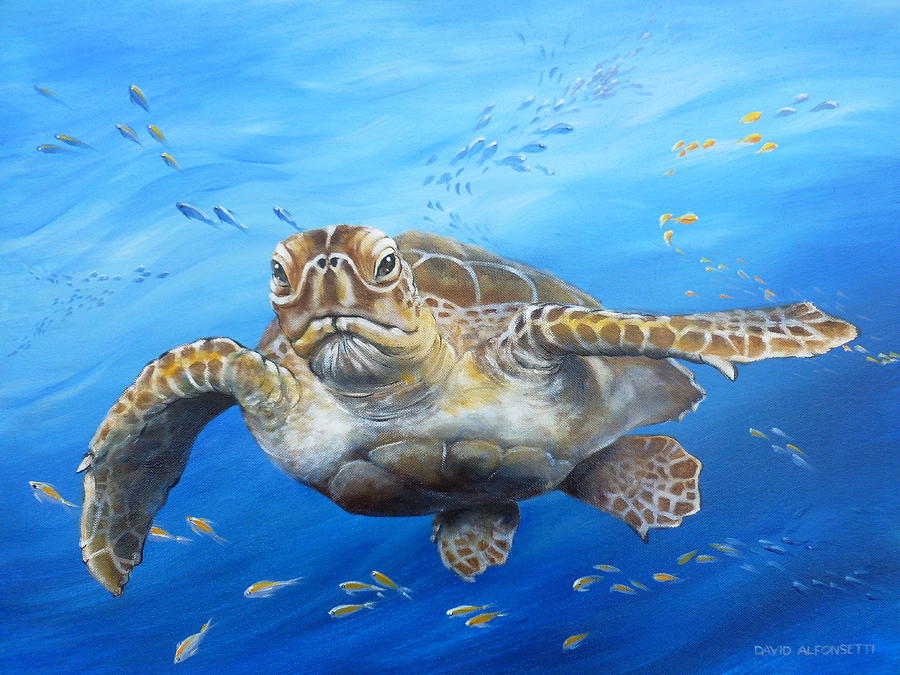This illustration by David Alphonsetti showcases a meticulously detailed sea turtle swimming underwater, prominently placed at the center of a blue ocean scene. The turtle, depicted from the front, features a richly textured shell with shades of brown and gold and well-defined scales interspersed with white skin. Its almond-shaped eyes and visible nostrils add to the realistic portrayal, alongside its wrinkly jaw. The turtle’s front flippers, which resemble large flippers covered in giraffe-like spots, are extended to the sides, with the left one slightly curved downward, and its smaller back paddles trail behind. Surrounding the turtle, schools of fish, including blue, yellow, gold, orange, and silver varieties, weave through the water, creating ribbon-like formations in the vibrant blue depths. The scene suggests daytime as light filters through the water from above. The artwork is signed "David Alphonsetti" in the lower right corner.